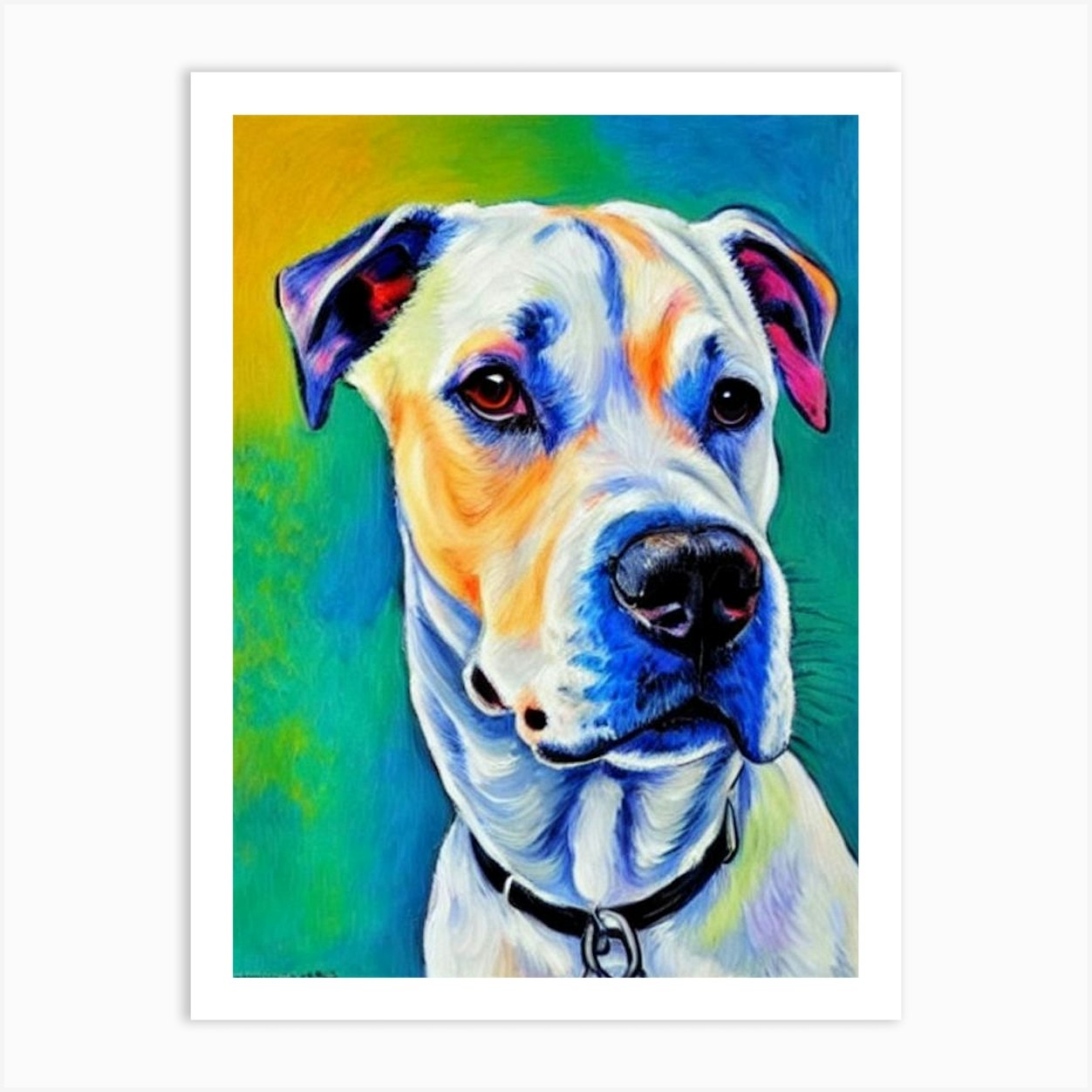This is a painting of a majestic Great Dane dog, prominently featuring its head and upper torso. The dog has predominantly white fur with a mixture of colors adorning its face and ears. The face is notably decorated with varied hues: its black snout and large brown eyes are framed by patches of orange and red, with blue and yellow highlights around the eyes and on the neck. The right side of its face includes a striking streak of bright red and orange, while the left ear is purple with black and red accents. The right ear’s interior exhibits pink and black tones with a bluish tinge. The dog's floppy ears, large nose, and expressive, slightly red eyes contribute to its dignified appearance. It also wears a black collar with silver links. The background of the painting transitions through an array of colors: it starts with blue and green at the bottom, moves to orange and yellow towards the top right corner, and reverts back to green and blue, creating a dynamic yet harmonious backdrop. The focal point of the artwork is the dog's direct, piercing gaze, making it both realistic and captivating.